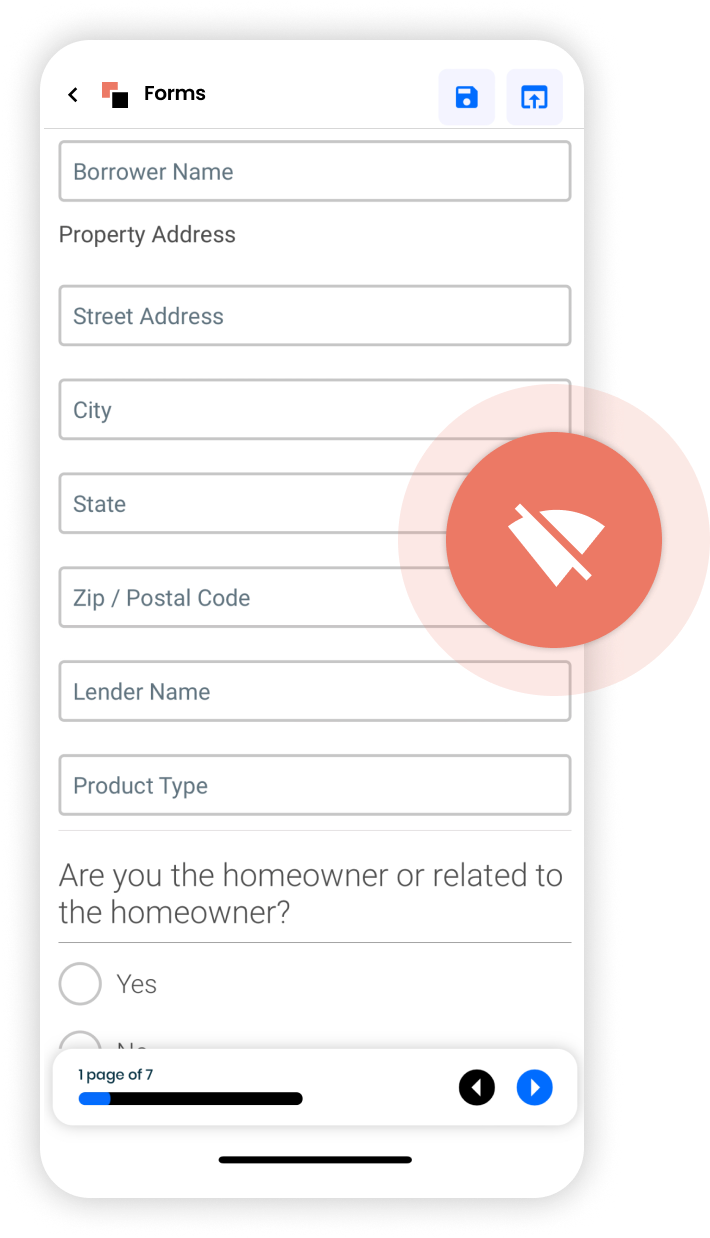The image depicts a digital form interface with multiple sections and various icons. 

1. **Top Left Section:**
   - A red circle with a slash through a Wi-Fi symbol indicates no connectivity.

2. **Main Form Details:**
   - Fields for borrower information, including:
     - Borrower Name
     - Property Address (sub-fields for street address, city, state, and ZIP/postal code)
     - Lender Name
     - Product Type
   - A question asking "Are you the homeowner or related to the homeowner?" with the option "Yes" selected, although the corresponding circle is not checked.

3. **Bottom Section:**
   - An indication that the form is loading, specifying "Page 1 of 7".
   - Navigation icons: a black circle with a left arrow, a blue circle with a right arrow.
   - A white smartphone icon.

4. **Central Focus:**
   - A prominent red circle in the center, slightly out of focus at the edges, emphasizing a Wi-Fi symbol with a slash mark, reinforcing the theme of no connectivity.